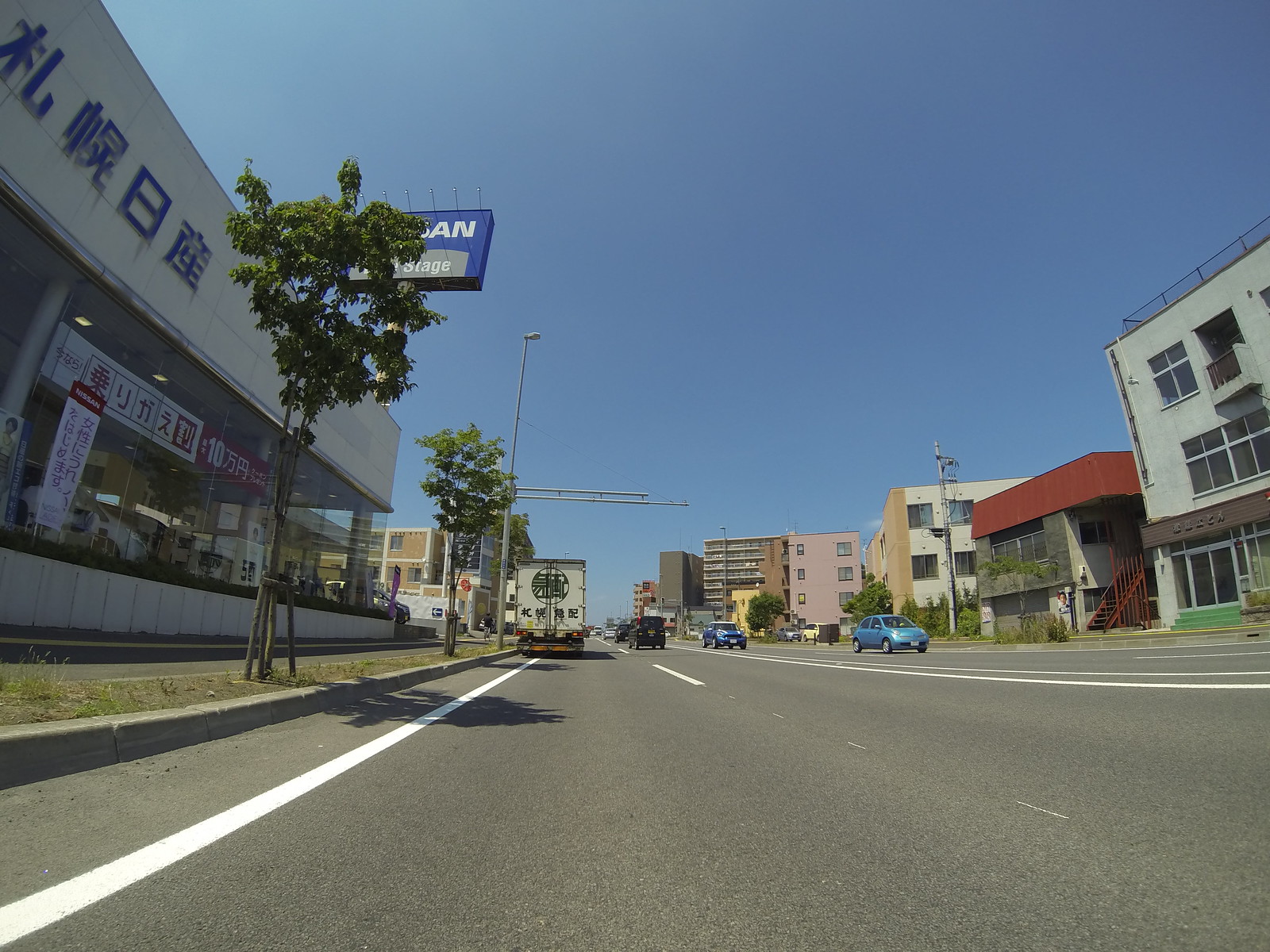This is a vibrant color photograph taken outdoors at ground level in a city setting, possibly from the perspective of someone lying down on the left side of a city street. The image captures an urban landscape with various buildings lining the opposite side of the street. Prominently featured is a storefront with a red roof, next to a taller, grayish, three-story building that also has storefront windows, though the contents are indiscernible due to the distance. On the left side of the street, a large storefront, which might be a car dealership, comes into view. It displays expansive windows typical of such establishments, and a portion of a blue sign is visible above, showing the letters "A-N". The rest of the sign is obstructed by a small tree planted adjacent to the street, adding a touch of greenery to the scene.